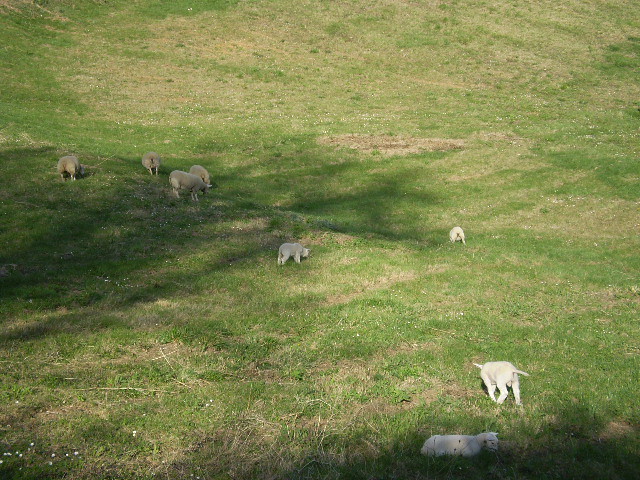In this vibrant color photo, we look down across rolling green hills adorned with patches of brown grass and tiny blooming white flowers in the bottom left corner. The pastoral scene is animated by the presence of sheep grazing peacefully. Along the bottom of the image, a prominent white sheep lies in a bit of shade, possibly chewing its cud, while another one, believed to be a ram, strides away from the camera with its tail held high. The foreground features a couple of young sheep, distinguishable by their recently sheared coats, contrasting with a group of adult sheep further up the hill, whose fuller wool fluffs in the sunlight, indicating they are ready for shearing. Shadows from tree limbs and branches frame the scene from the left, creating a picturesque play of light and shadow on the rolling pasture.